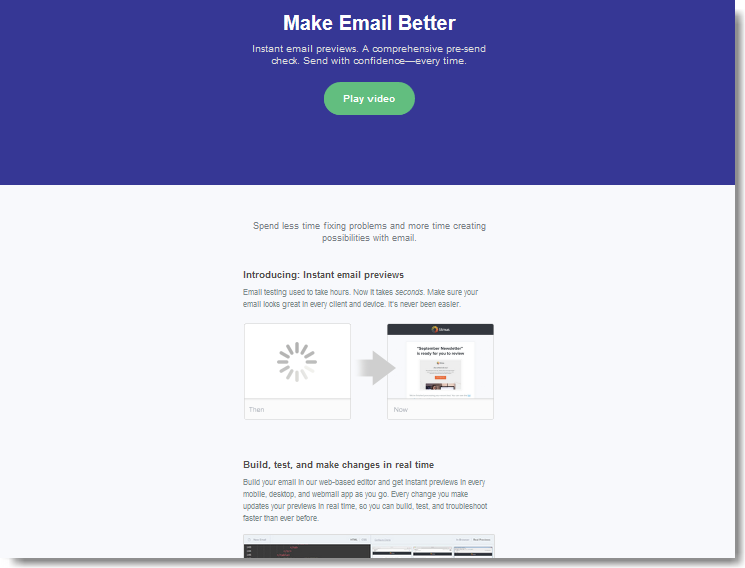**Web Page Screenshot: Enhancing Email Efficiency**

The top banner, in a purplish hue, prominently displays the text: "Make Email Better." Below this headline, the page introduces a feature with a detailed description: "Instant email previews, a comprehensive pre-send check. Send with confidence every time." 

A green "Play Video" button is situated beneath this introductory text. 

The next section of the page is primarily white with a light gray backdrop. It features a compelling proposition: "Spend less time facing problems and more time creating possibilities with email. Introducing instant email previews."

Following this, a video titled "Then and Now: Introducing Instant Email Previews" is embedded in the section. While some of the text around this video is not completely readable, the gist is clear: "Build, test, and make changes in real-time."

In summary, the web page is designed to boost email efficiency. It highlights the benefits of instant email previews, offers a pre-send checking system, and provides two informative videos illustrating the features and process.